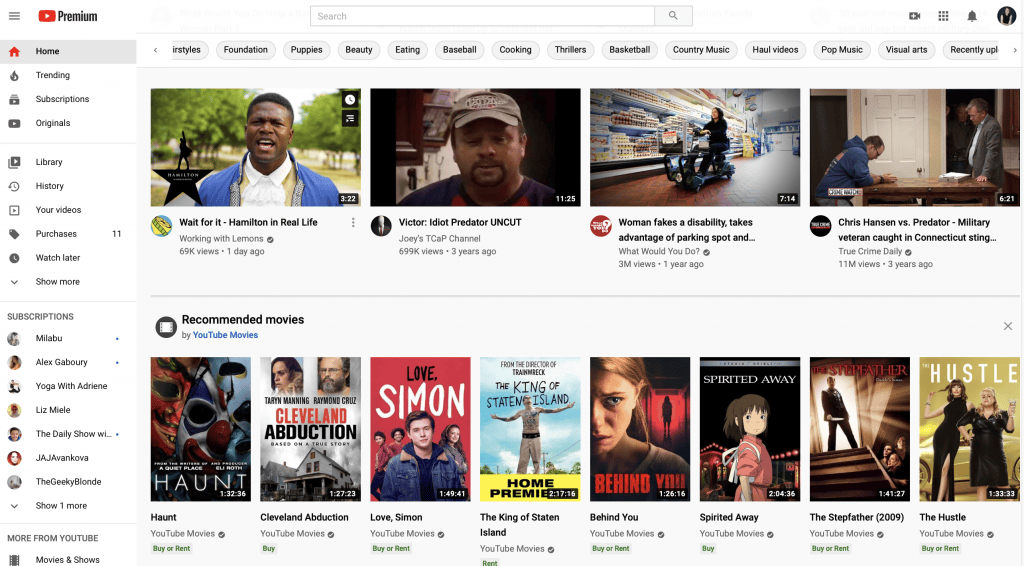This image showcases the YouTube Premium interface, set against a sleek white background. In the top left corner, there are three short, black horizontal lines, approximately a quarter of an inch in length. Adjacent to these lines is the Google Red Play button in black, labeled "Premium." At the center of the screen is a long, rectangular search bar featuring a light blue section on the right end with a black search icon.

On the right side of the interface is a profile picture depicting an individual wearing a black shirt, followed by a notification bell icon, a grid of nine dots (three across and three down), and a black camera icon with a white plus sign within it.

On the left side of the screen is a vertically arranged list of clickable options, each accompanied by their respective icons. The first option displays a red home icon followed by the word "Home" in black. Next, there's a fire icon for "Trending," and then "Subscriptions" appears multiple times. A thin gray line divides this list, below which six more items are listed, followed by another thin gray line. At the bottom, it says "Subscriptions," showing six names with an option to "Show one more."

Across the top of the screen are various clickable gray buttons for different video categories. The first button is partially cut off and appears to say something like "styles." Following that, buttons for "Foundation," "Puppies," and "Beauty" are visible, with around twelve categories in total.

Below these buttons, four video thumbnails are displayed, each with the video's title, upload time, and view count. Further down, after another thin gray line, there's a section titled "Recommended Movies" in black. Below this heading, "YouTube Movies" is written in blue text. This section showcases eight movie covers, each with the movie's title underneath and options to rent or buy.